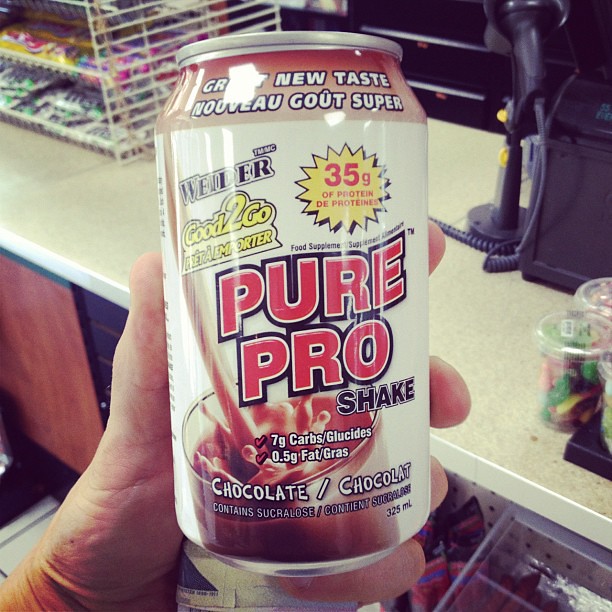The image features a close-up shot of a person's hand holding a can of Pure Pro Shake prominently in front of the camera. The can, centered and taking up most of the frame, is labeled as chocolate-flavored, boasting 7 grams of carbs, 0.05 grams of fat, and contains sucralose. The can has a volume of 325 milliliters and is marketed with the tagline "Good to Go" and "Great New Taste." In the background, a secondary image shows the shake being poured into a glass, with the liquid splashing up, enhancing the appeal and freshness of the product. The setting appears to be a store checkout counter, adding a realistic context to the scene.